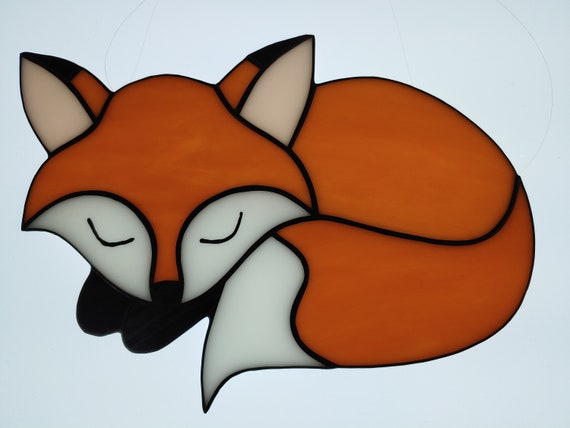This image portrays a beautifully detailed, artistic depiction of a sleeping fox, reminiscent of stained glass artwork. The fox, characterized by vivid orange panels, features textured variations that evoke the appearance of real glass. Its face and body are bordered by bold, black outlines, typical of stained glass art. The curled, sleeping fox showcases distinct features with white inner ears, white patches around its eyes, and the white tip of its otherwise orange tail. The fox's paws and the backs of its ears display black tips, adding to the contrast. In addition to these primary colors, light shades of cream and sky blue add depth, particularly noticeable in the eye patches and tail tip. The background is predominantly white, enhancing the fox's vibrant colors. Though subtly visible, thin wires seem to support the piece, contributing to its stained glass window-like appearance. Despite the absence of direct light or text, the fox artfully rests in a serene, curled position, with delicate arches above its closed eyes, all against a simple, elegant white canvas.